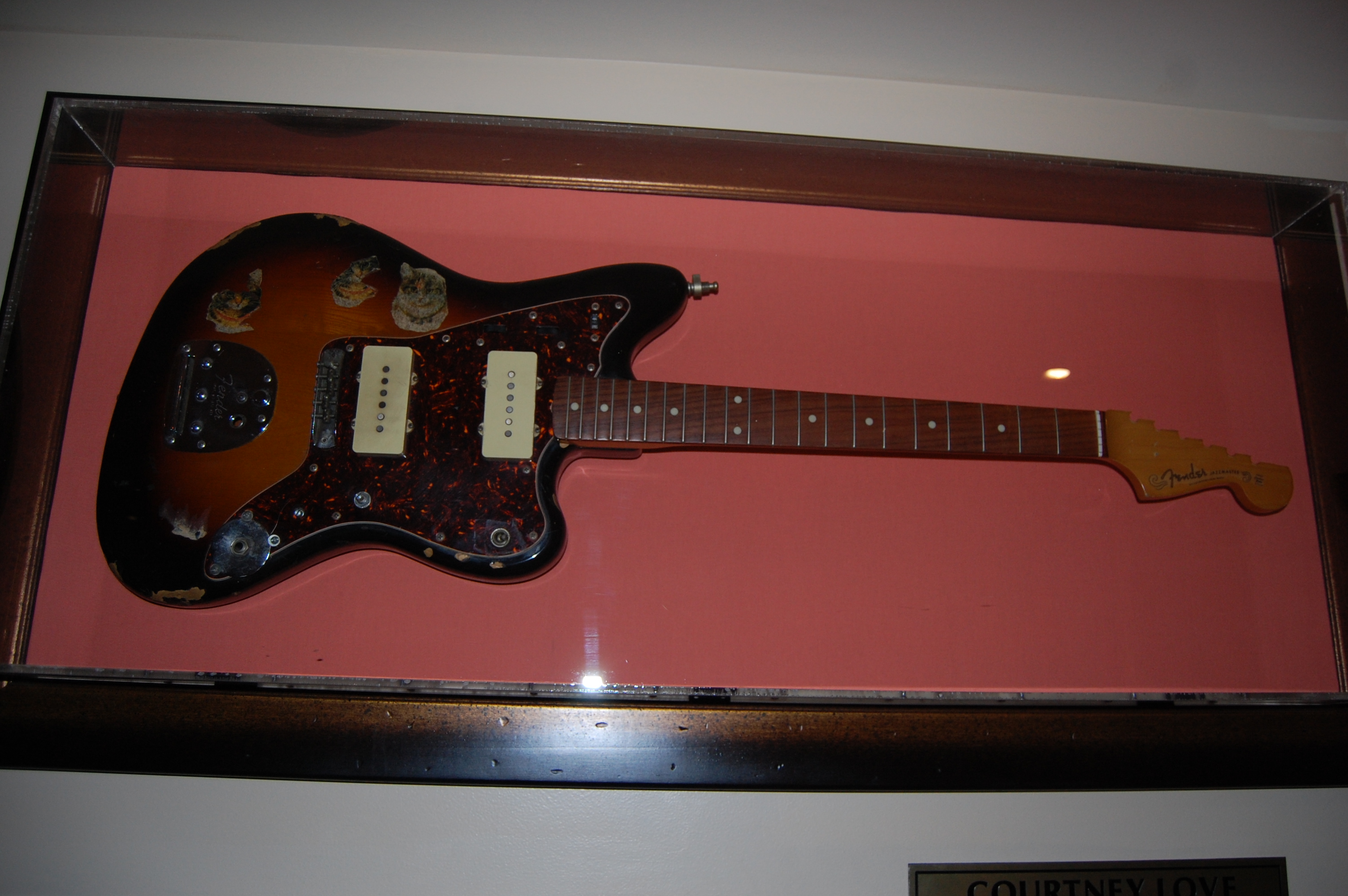The image depicts an electric guitar mounted within a wooden frame that hangs on a white wall with a white ceiling visible where they converge, suggesting a gallery or possibly a home exhibit. The frame is rectangular and made of brown wood, and it encloses a pink background. The guitar itself features a dark wood grain shaft, with white fret dots, leading up to a lighter wood area where the tuning pegs would typically be, although they are absent in this display. The guitar body exhibits a combination of dark black, red, and orange hues, with its distinct shape and the jack input for an amplifier clearly visible. The overall appearance of the guitar suggests it may be vintage and significant, accentuated by its presentation in a dedicated frame.